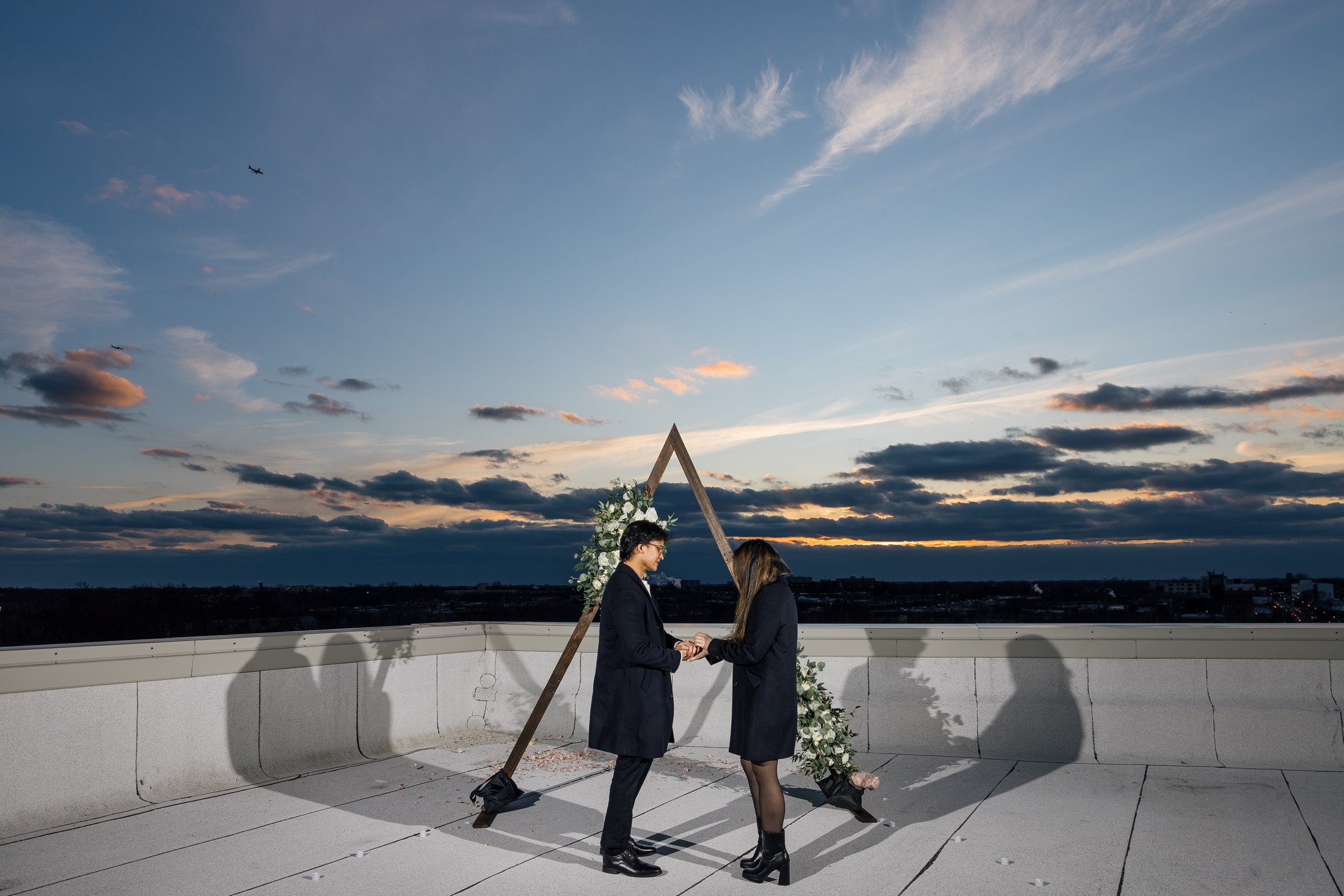This color photograph, in landscape orientation, depicts a young couple in their late 20s to early 30s standing on a rooftop patio during sunset, likely celebrating an engagement or wedding. The couple stands in the center of the image, facing each other and holding hands, beneath an upside-down V-shaped boho arch adorned with flowers—a garland at the apex and a spray of white flowers climbing the right leg. They are both dressed in black; the woman wears a knee-length black dress with black boots and long dark hair, while the man wears a black overcoat, black trousers, and black shoes. The white-tiled patio, edged by a low stone wall, reflects the soft, ambient light of the descending sun. The sky is a striking tableau of gradient blue with streaks of yellow, pink, and orange hues beneath dark gray clouds, hinting at the approaching dusk. This serene, romantic moment is accentuated by strong shadows cast on the ground, suggesting the presence of a bright light source, likely from the person taking the photograph.